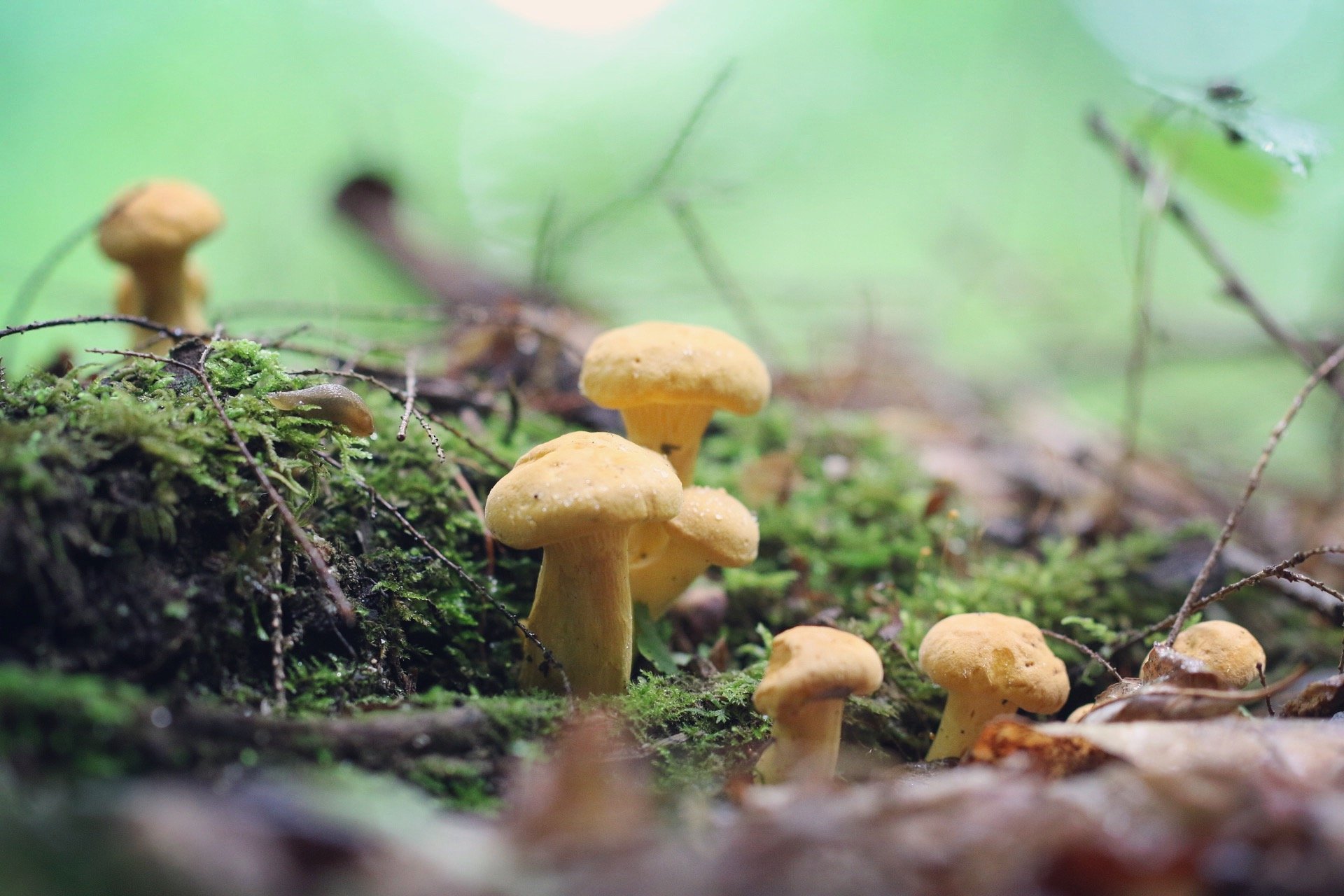This horizontal, ground-level photograph captures a detailed close-up of a cluster of six to seven yellow toadstools, sprouting from a lush, green mound of dirt covered with leaves and short grass. The composition emphasizes the pale yellow mushrooms with their smooth, uniformly colored stems, some tall and prominent, while others are significantly smaller. In the foreground rests a log, with a few toadstools peeking over it, and others, particularly taller ones, receding into the back. The blurred background, a canopy of light green vegetation, provides a soft contrast and keeps the viewer's focus firmly on the vibrant toadstools. There is an indistinct shape behind the taller toadstools that could be a bird or another log, adding an element of mystery to the scene. The overall atmosphere is damp and lush, indicative of a moist, forest floor setting during daytime.